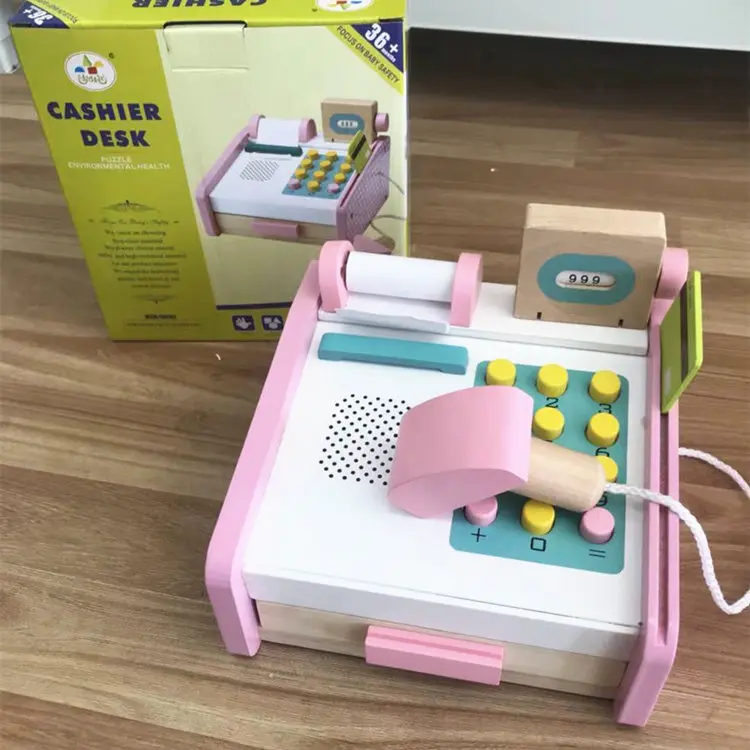This detailed image showcases a child's wooden toy cash register prominently positioned on a wooden floor. The cash register itself is pink on the sides, featuring multiple round buttons in yellow and pink hues on a green number pad. It boasts a built-in block drawer that can be pulled out, a roll of white receipt paper on the top left, and a number counter displaying "999" at the top. The sides of the register have a groove where a wooden credit card is currently slid in. Holes on the register suggest a speaker, and behind it hangs a white string connected to a round metal object. In the top left corner of the image stands the toy's cardboard box, predominantly green, displaying an illustration of the cash register and labeled with text such as "Cashier Desk," "Puzzle," and "Environmental Health." There are no other objects in the image, and the clean wooden floor and absence of other furniture indicate it could be in a room like a bedroom or a kitchen.